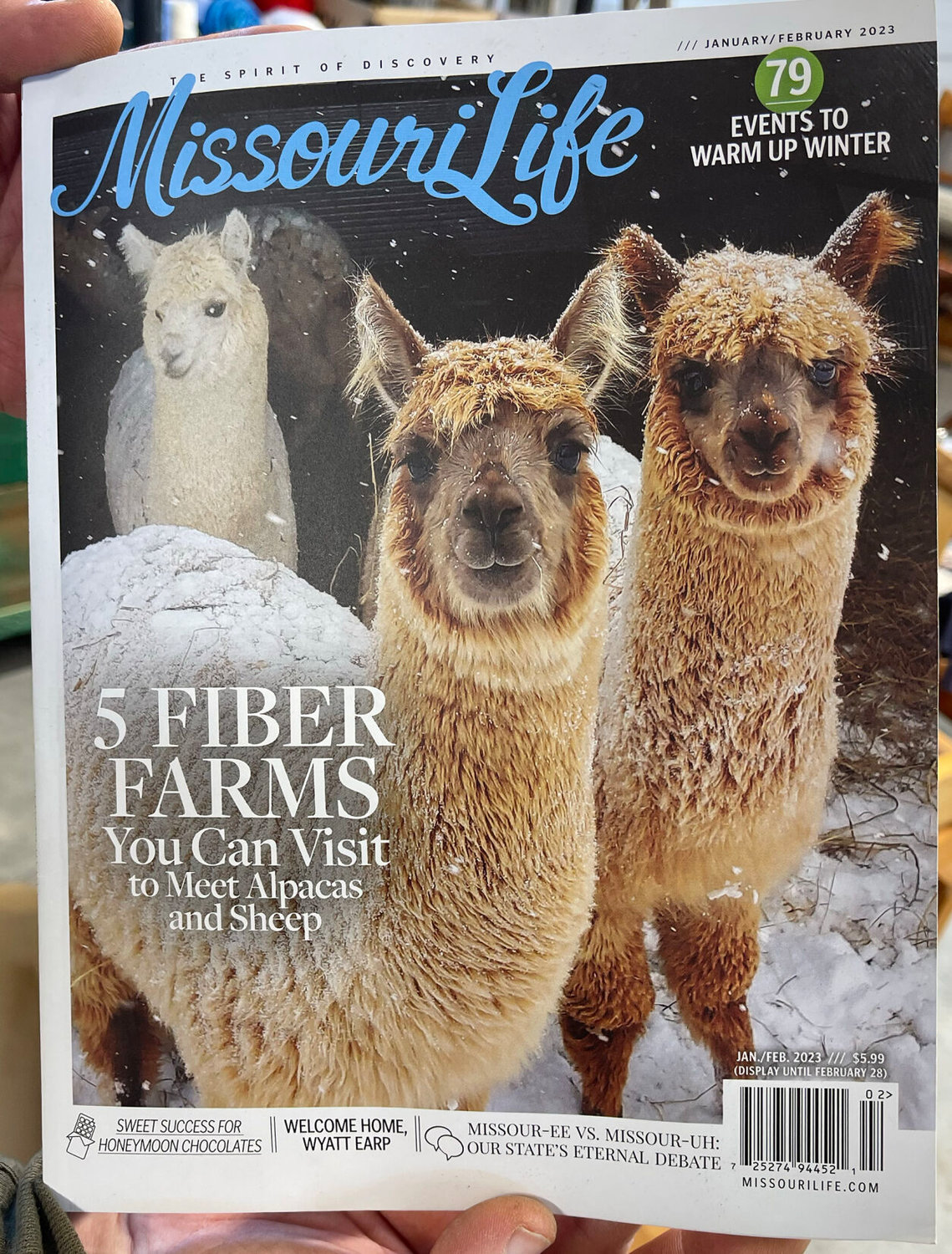The front cover of the January-February 2023 issue of Missouri Life magazine, held by a hand at the edges, prominently features the title "Missouri Life" in blue script on a dark brown background, along with the tagline "The Spirit of Discovery." Three alpacas are pictured amidst a snowy landscape, with snow delicately covering their fur and noses; two are ginger-colored and positioned in the front, while one predominantly white alpaca stands slightly behind them. The scene denotes a light snowfall with snow settled on the ground and on some dried brown brush. Text across the cover includes headlines such as "79 Events to Warm Up Winter," "Five Fiber Farms You Can Visit to Meet Alpacas and Sheep," "Sweet Successes for Honeymoon Chocolates," and "Welcome Home Wyatt Earp." Additionally, there's a teaser for an article on Missouri's eternal debate: "Missouri vs. Missoura." The magazine, priced at $5.99, is to be displayed until February 28th, 2023, as indicated by the UPC label.